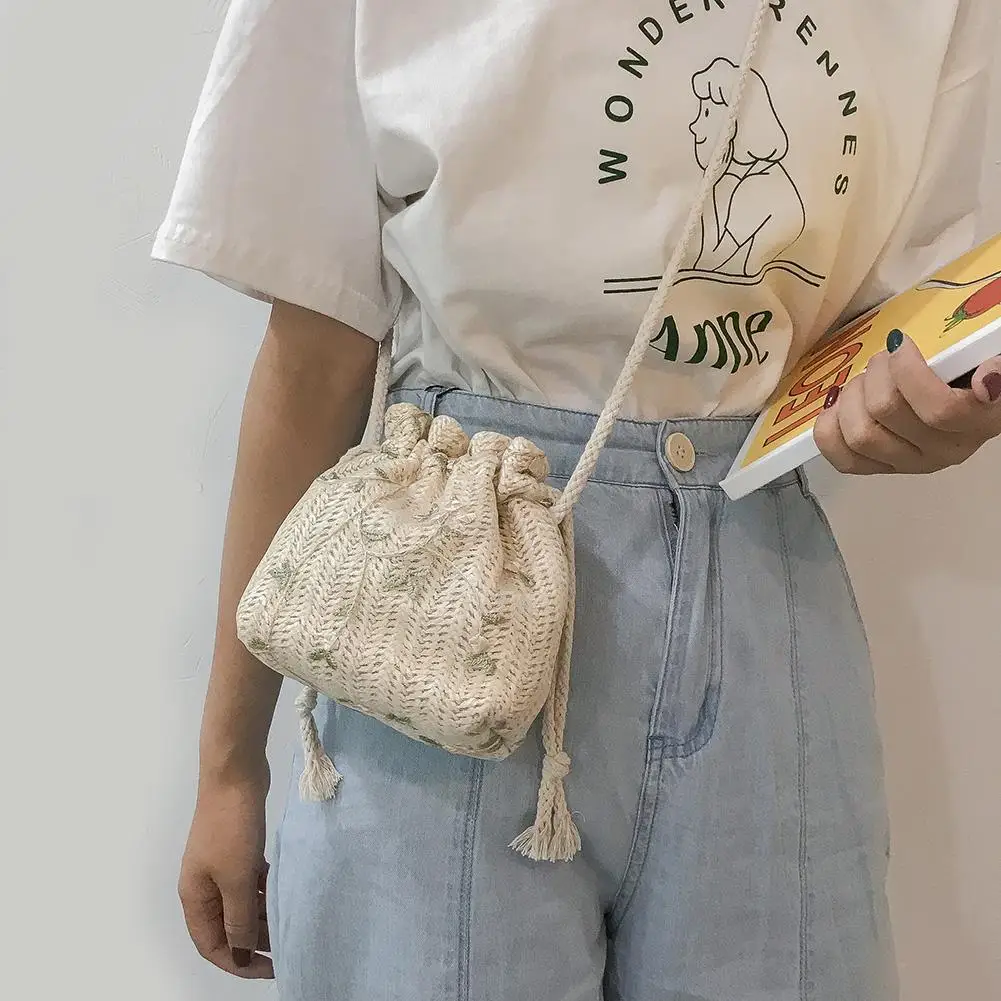The image depicts a young woman standing against a dual-colored wall, with the left side light blue and the right side gray. She is wearing blue jeans paired with a large white t-shirt featuring the text “Wonder Rene's Anne” along with a simple graphic of a girl with short hair seated at a desk. The t-shirt has half sleeves, and the woman appears to be dressed in retro or vintage attire. She holds a yellow-covered book with the word "Leon" in her left hand, and her nails are painted plain black. Draped across her body is a cream-colored, crocheted handbag adorned with a floral or leaf pattern and fringe, which hangs from a rope-like strap. The high-waisted jeans have an elastic waistband with a button and zipper closure. The setting and outfit suggest a fashion photo shoot.